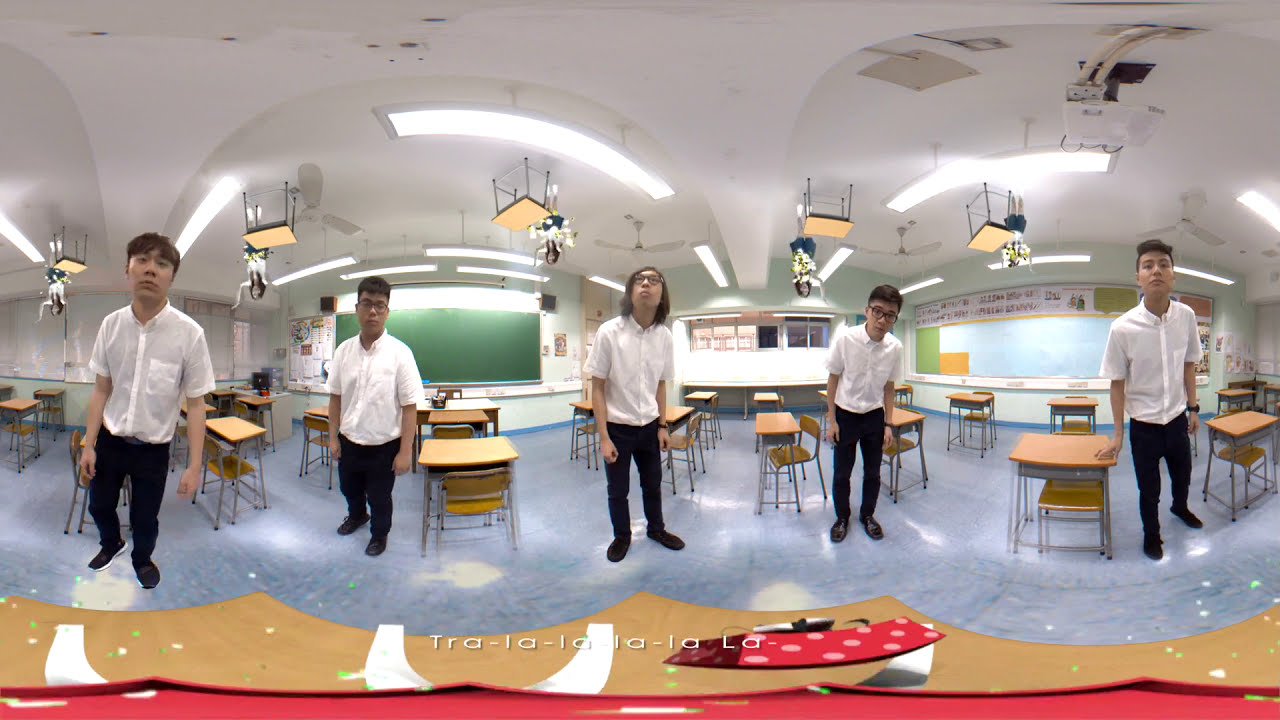The image depicts a surreal, panoramic view of a well-lit classroom, enhanced by VR and 360 camera effects. The classroom features a light blue floor and scattered student desks, creating a conventional school setting at ground level. However, the scene takes an odd twist with desks and chairs appearing to hang upside down from the ceiling, where people are also seated, suggesting a duplicated and disorienting effect. Five Asian men, dressed uniformly in white short-sleeved button-up shirts, black pants, and black shoes, are positioned in the foreground, clearly visible and all facing the camera. The men on either end look directly at the camera, while the central figure looks upwards toward the ceiling. The background shows a green chalkboard, contributing to the classroom ambiance. Text reading "tra la la la la la" is displayed at the bottom of the image. The fisheye lens effect further distorts the composition, presenting a fragmented vision where elements from the three images blend into one another, featuring partially visible chairs and an overall surreal aesthetic.